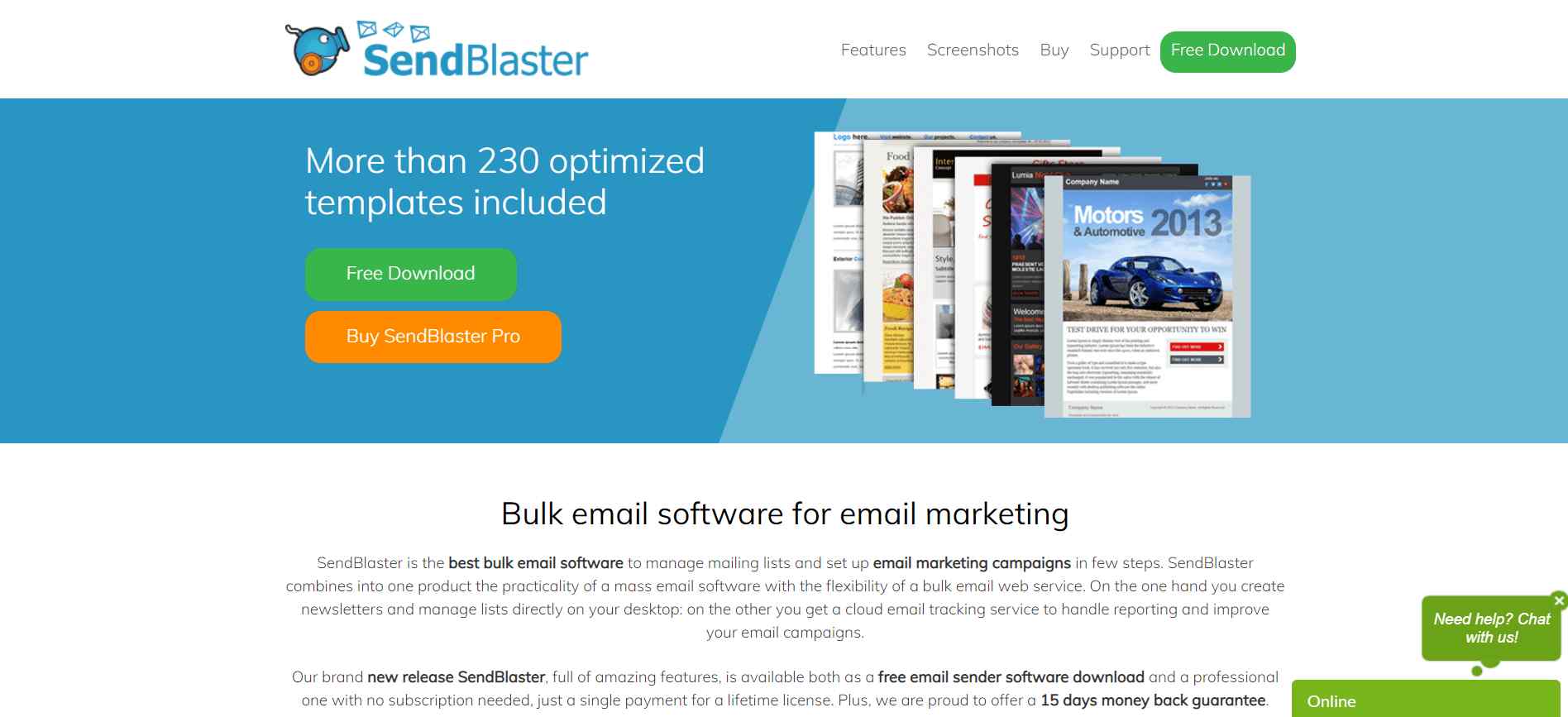The image showcases a web page with a clean white background. In the top-left corner, there is a distinctive blue icon resembling a cannon or mailbag, with a hint of orange at its base. Three white envelopes with blue borders are emerging from this icon, situated above the company name. "Send" is displayed in bold blue text, followed by "Blaster" in regular font.

To the right of the logo, the navigation menu items "Features," "Screenshots," "Buy," and "Support" are listed in black text. Adjacent to these, there is a green, rounded button with white text reading "Free Download."

The upper section of the page features a blue-to-light-blue gradient background divided diagonally. On the left side, white text reads "More than 230 Optimized Templates Included," accompanied by another green "Free Download" button. Below this, there is an orange button with white text that says "Buy Send Blaster Flow Pro."

In the center of the page, there are several images depicting different web pages. Underneath these images, black text declares, "Bulk Email Software for Email Marketing," followed by smaller fine print content that is not legible.

In the bottom right corner, there is a green box with white text reading "Online," and above it, a green chat bubble with the message "Need Help? Chat with Us" in white text.